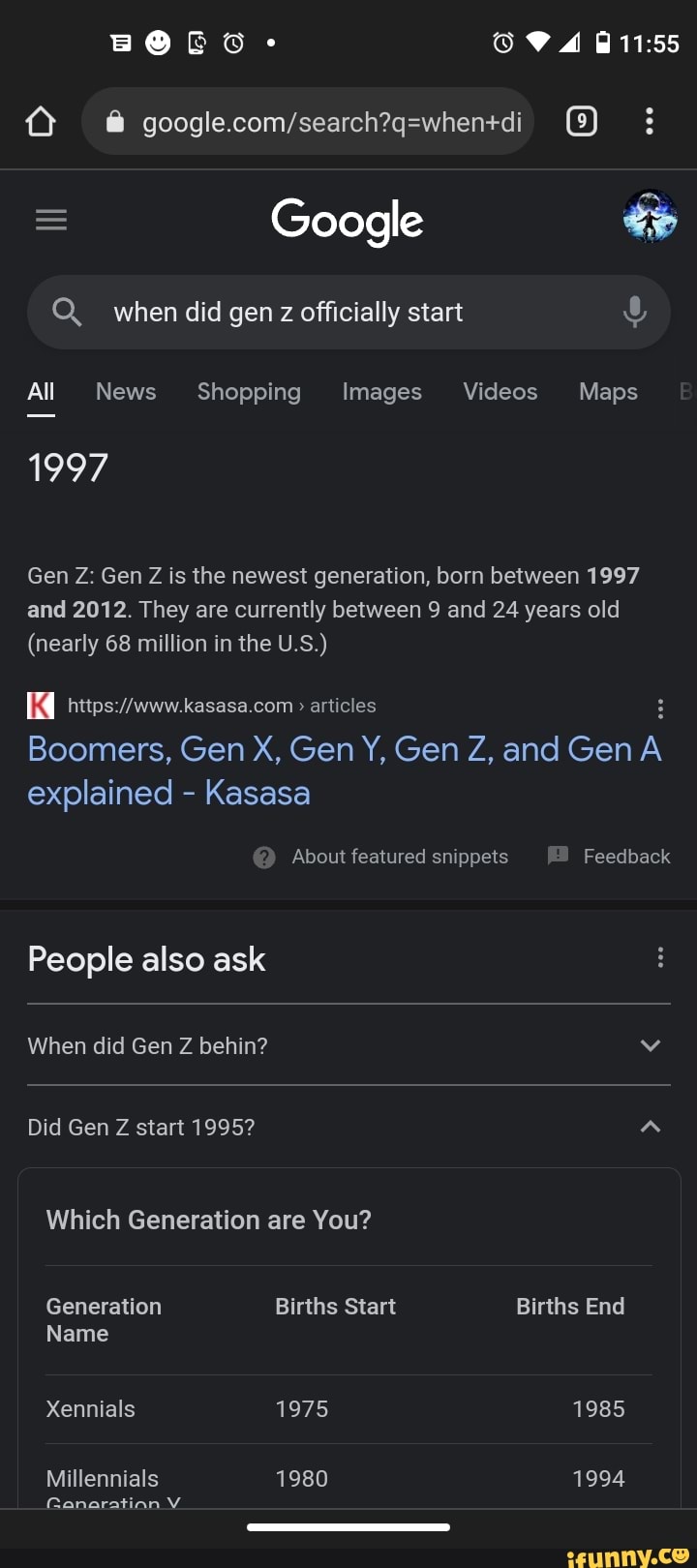Here is the cleaned-up and detailed descriptive caption for the image:

---

The image shows a smartphone screen displaying Google search results. At the top of the screen, the status bar includes several icons: a speech bubble, a happy face, a phone with a refresh icon, an alarm, Wi-Fi signals, and a battery icon showing half a bar of charge. The clock reads 11:55 AM. 

Beneath the status bar, the URL reads "google.com/search," and there are nine tabs open in the browser. The recognizable Google logo appears below this, above a search field containing the query, "When did Gen Z officially start?"

The search results are categorized into tabs: "All," "News," "Shopping," "Images," "Videos," and "Maps." Under the "All" category, the primary result states, "1997. Gen Z is the newest generation, born between 1997-2012. They're currently between 9 and 24 years old, nearly 68 million in the US," accompanied by a link to an article on kasasa.com.

There are also related questions listed under "People also ask," including: 

- "When did Gen Z begin?"
- "When did Gen Z start? 1995?"
- "Which generation are you?"
  
A table lists generations with their birth start and end years, such as:

- Xennials: 1975-1985
- Millennials: 1980-1994

In the bottom right-hand corner of the screen, the ifunny.co logo is visible. In the upper right-hand corner, next to the Google logo, there's a user icon resembling a cartoon image. 

---

This caption provides a thorough description of the image and the information presented on the smartphone screen.